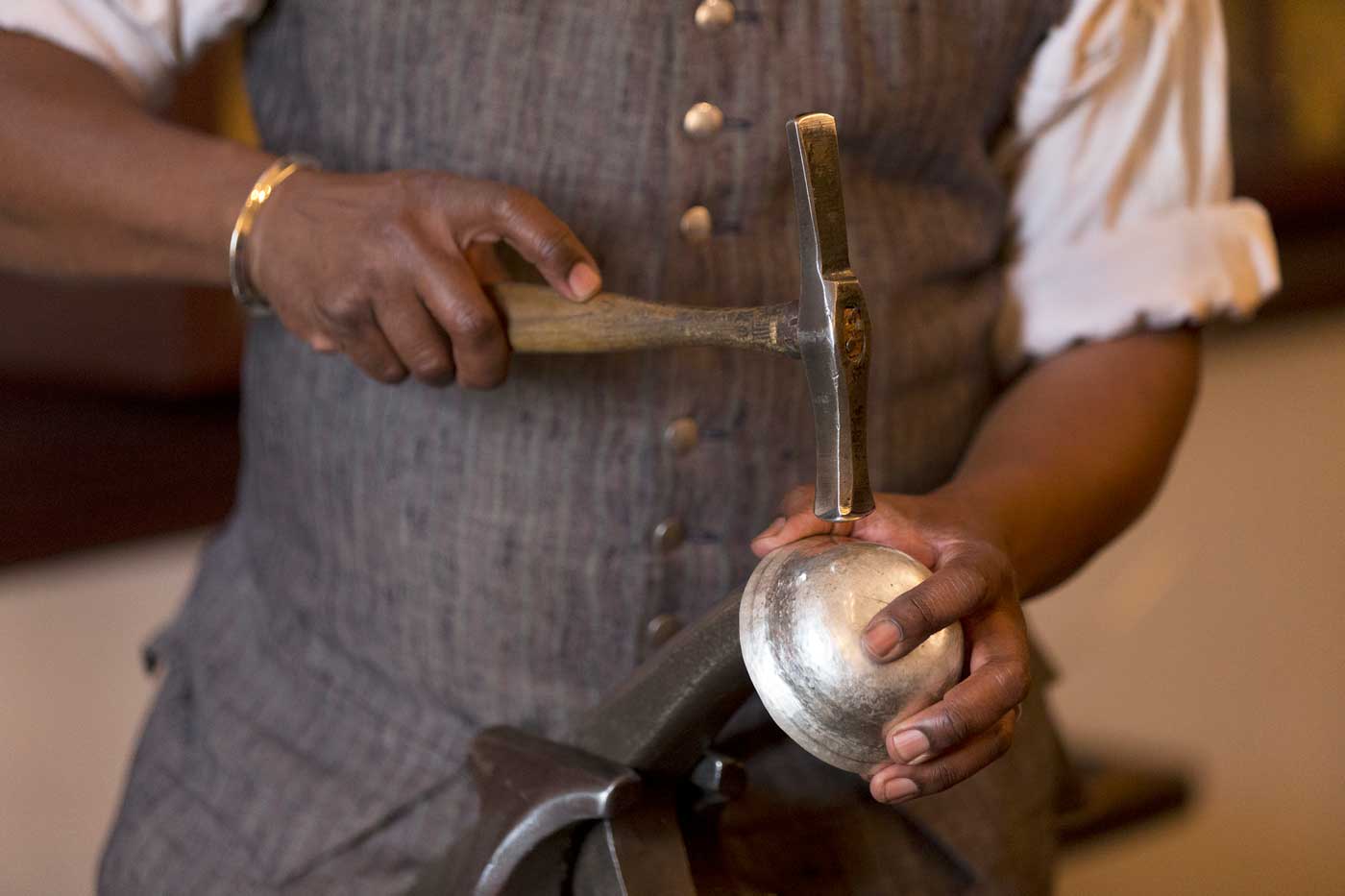In the image, we see a black man engaged in old-world metalworking, captured from below the neck to about his waistline. He is wearing a gray, buttoned jacket over a white shirt with its sleeves rolled up to his elbows, and gray pants. On his right wrist, he sports a gold-like bracelet. His right hand grips a long-handled hammer, distinguished by a thin, rectangular, metal head with a flat front and back. He's holding a rounded, silver metal object, resembling the top portion of a bell or a bowl, in his left hand. This object is positioned atop a black anvil or anvil-like machinery below him. The scene reflects a meticulous moment of shaping the metal using traditional methods.